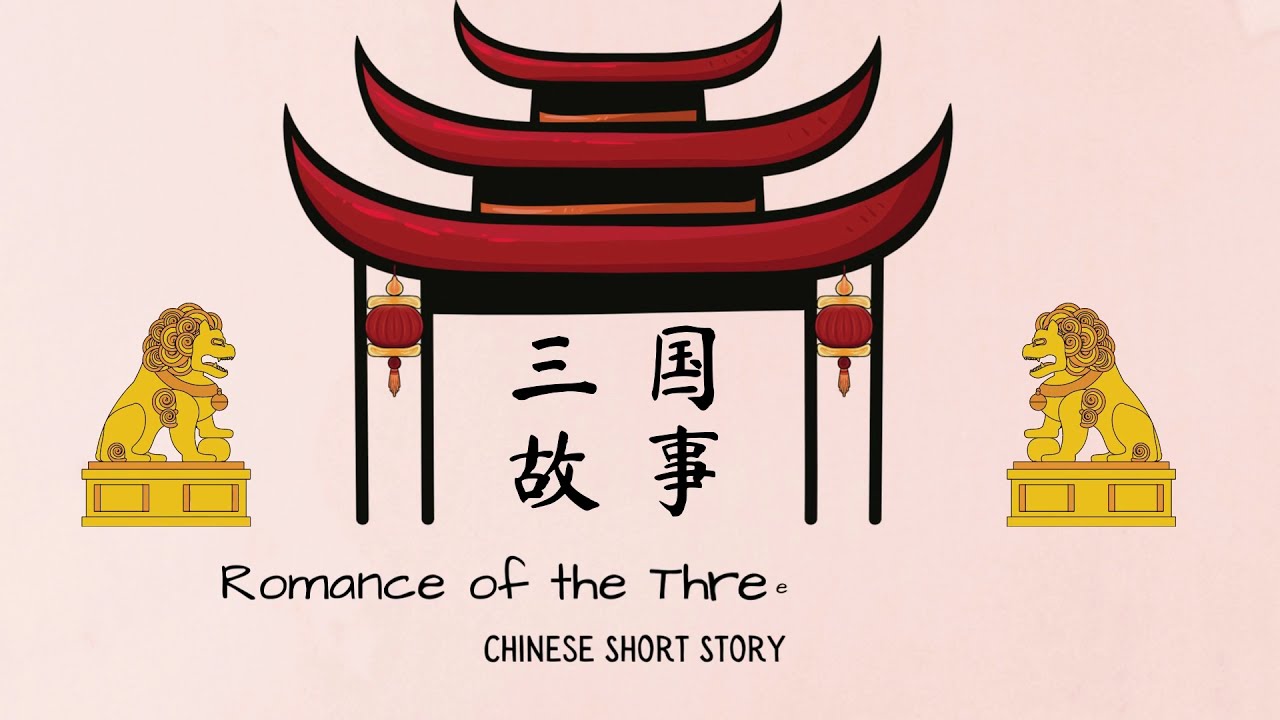The image appears to be promoting a performance or perhaps serving as a book cover, featuring a soft light pink background. Dominating the center is a detailed drawing of a traditional red pagoda-like structure with a three-tiered roof that curves and spikes upward at each level, each tier smaller than the one below it. Flanking this structure are two gold lion statues, both positioned in profile on raised rectangular platforms with orange trim. Each lion has curly hair and an orange collar with a bell, with one paw resting on a ball. The pagoda features red lanterns with gold trim hanging from two black pillars on either side, and the center includes black Chinese characters. At the bottom in bold black letters, the text reads: "Romance of the Three: Chinese Short Story."